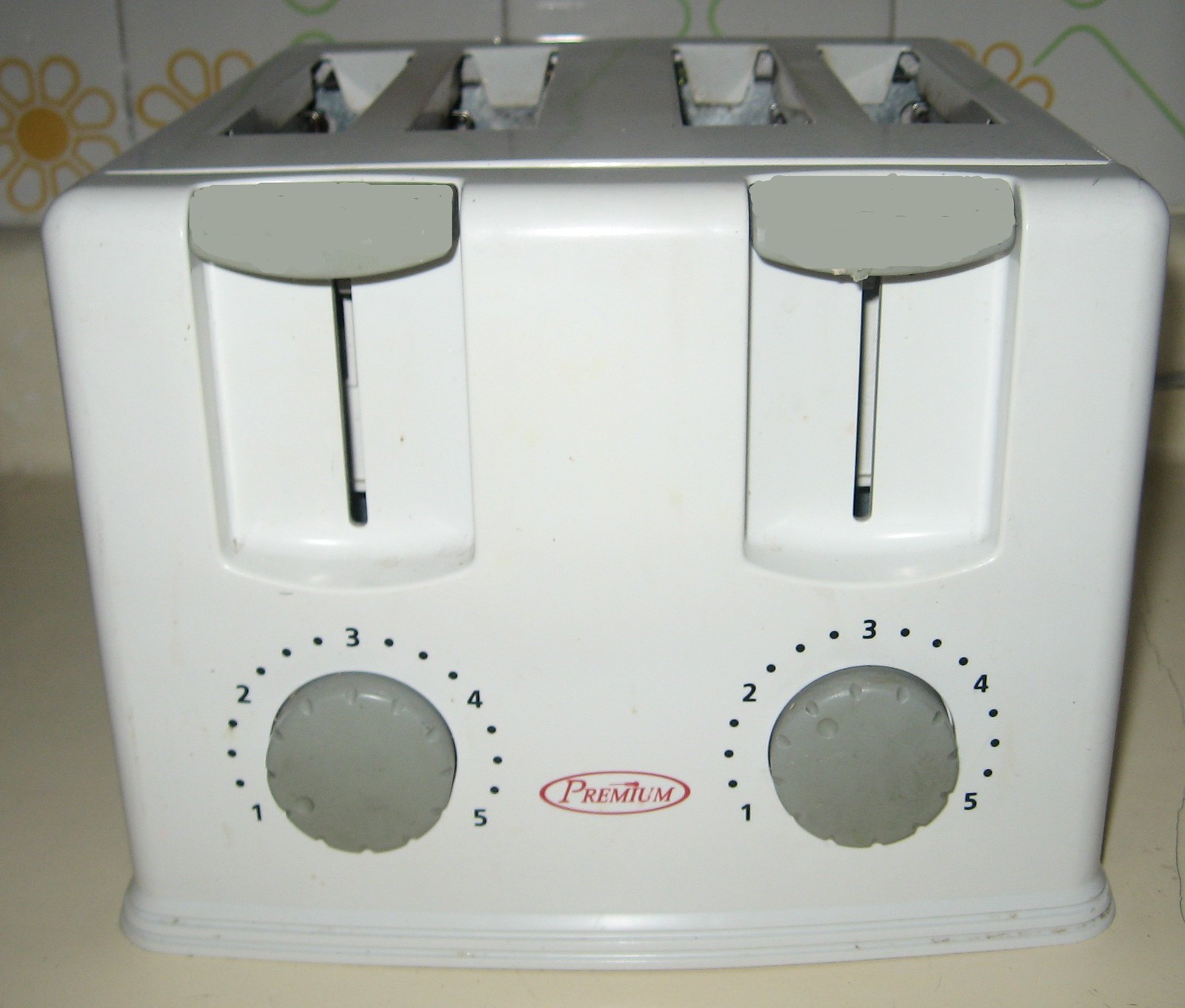This is a color photograph of a large, old-fashioned, white toaster with a blocky design, capable of toasting four slices of bread simultaneously. The toaster features four slots, divided into two pairs: two on the left and two on the right. Each pair has its own lever mechanism for lowering and raising the toast, allowing for separate controls. Below each pair of slots is a gray dial numbered from 1 to 5, with additional sub-level dots for fine-tuning the browning setting. The brand "PREMIUM" is visible in red print within an oval. The toaster is situated on a tan-colored kitchen counter, and the background features white wallpaper adorned with yellow floral patterns.